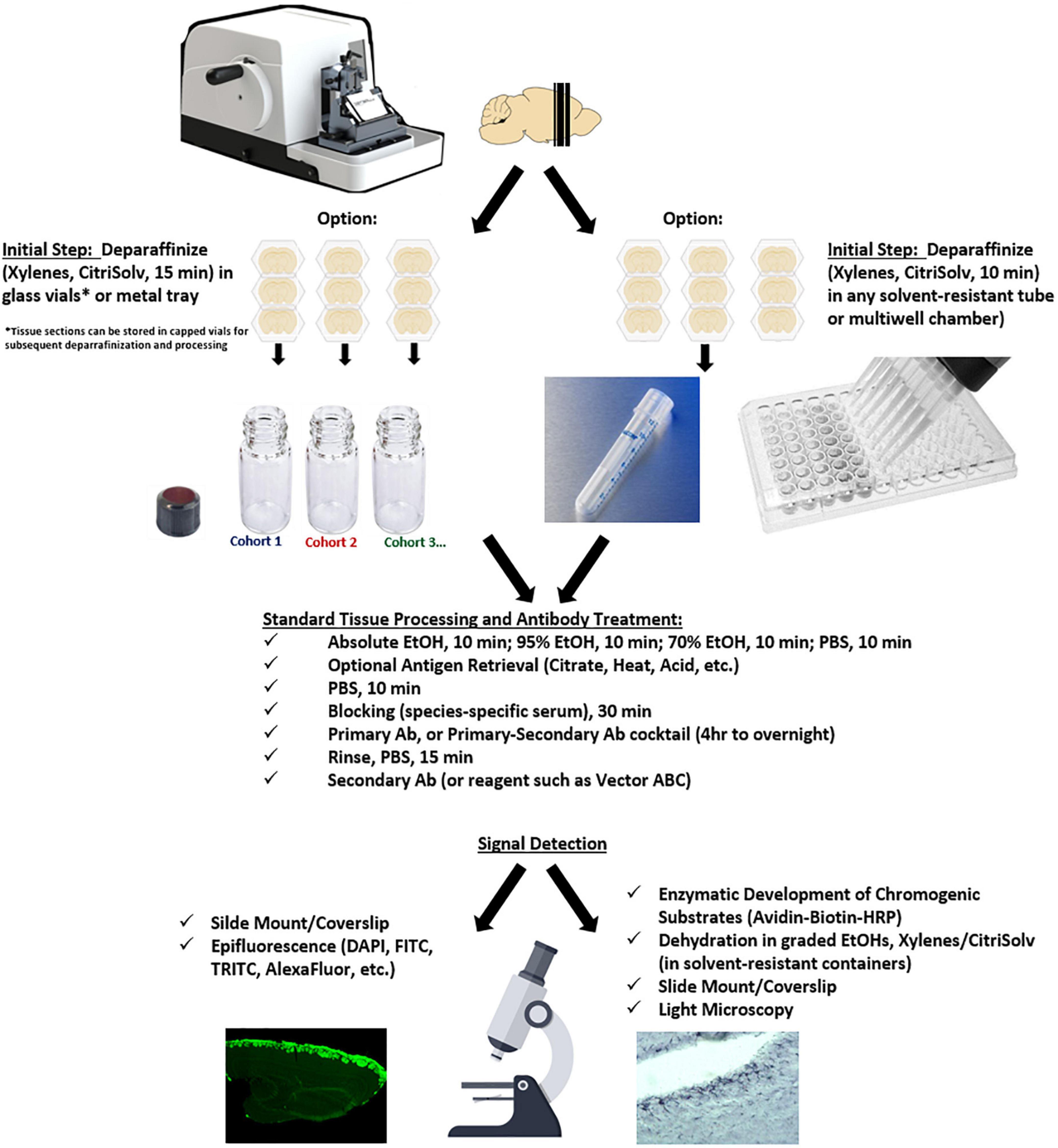The image features a detailed schematic against a plain white background, illustrating a scientific procedure, likely related to a medical or laboratory treatment involving tissue processing. At the top left, there is a white device with a black base and handle, and a gray metal portion in front. Adjacent to the right is an image of a brown brain with matter appearing to emanate from it. Black arrows direct the viewer's attention downward to a section labeled "Initial Step," which includes instructions on deparaffinization. 

The text describes the use of "xylene or Citrusol" for "15 minutes in glass vials or metal trays," with a note indicating that "tissue sections can be stored in capped vials for subsequent deparafinization and processing." To the right, alternative options are presented, showing different caps and bottles labeled as "cohort one, two, and three." 

A similar instruction is repeated, highlighting "deparaffinize, xylene, Citrusol, 10 minutes in any solvent-resistant tubes or multi-well chamber," supplemented by illustrations of tubes fitting into small circular holes. Further arrows guide the flow to a section on "Standard Tissue Processing Antibody Treatments," marked by a row of check marks listing various processes and treatments.

Continuing down, the diagram addresses "Signal Detection," with more arrows pointing to text and microscopic images displayed on the left and right. The bottom part of the image features close-up pictures presumably taken from a microscope, along with more medical-related text, reinforcing the methodological steps and procedural details.